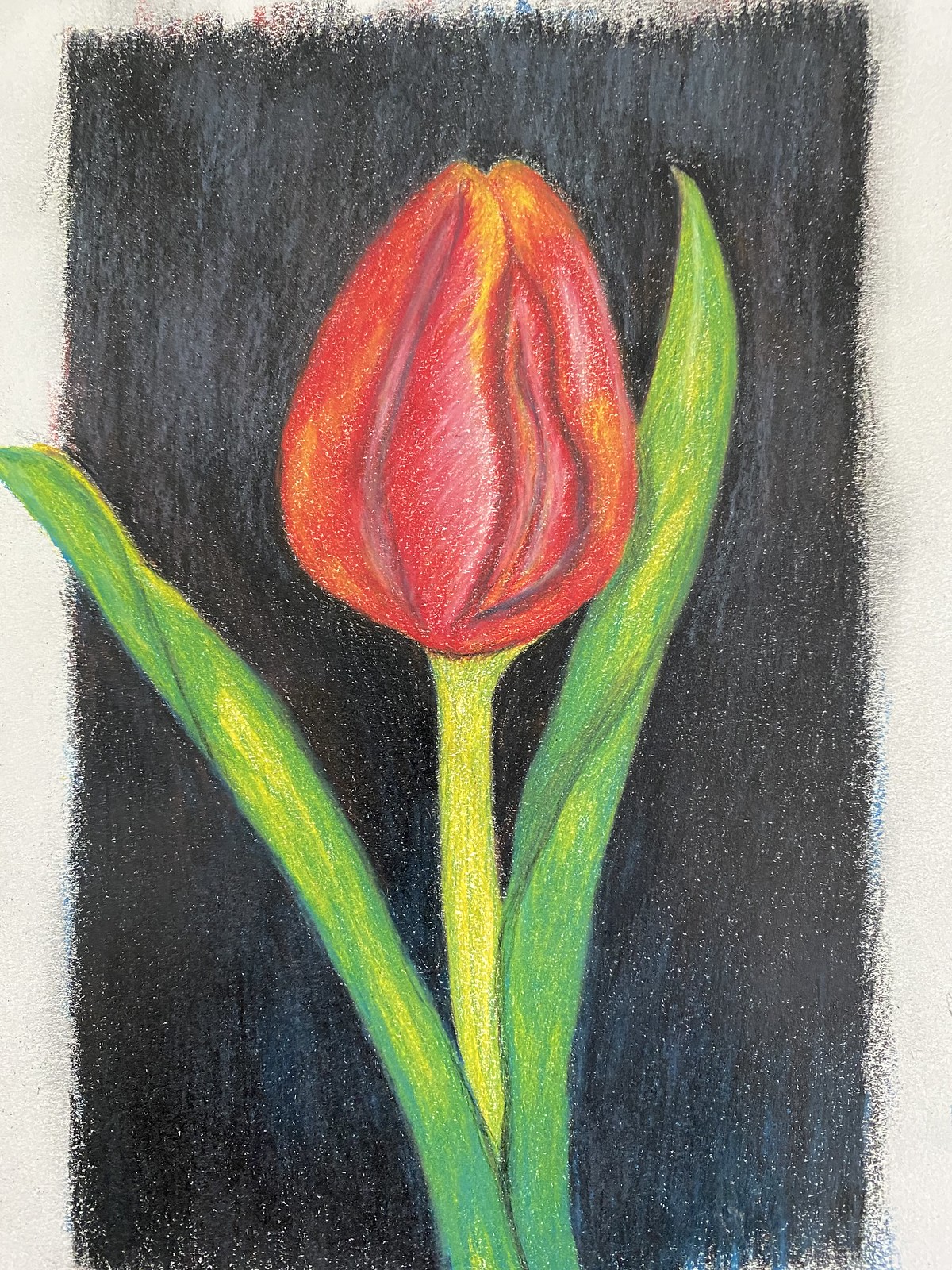This image showcases a meticulously crafted sketch done in marker, featuring a captivating flower against a deep black background. The illustration is framed by a distinctive gray-white border. The flower itself is detailed with two variegated leaves, one yellow and one green, providing a vibrant contrast. At the heart of the composition, a yellow stem supports a tightly closed red bud, reminiscent of lips poised for a kiss. The red bud is subtly accented with touches of yellow, adding depth and emphasizing its form. Though unsigned, the striking drawing stands out for its bold use of colors and intricate details.